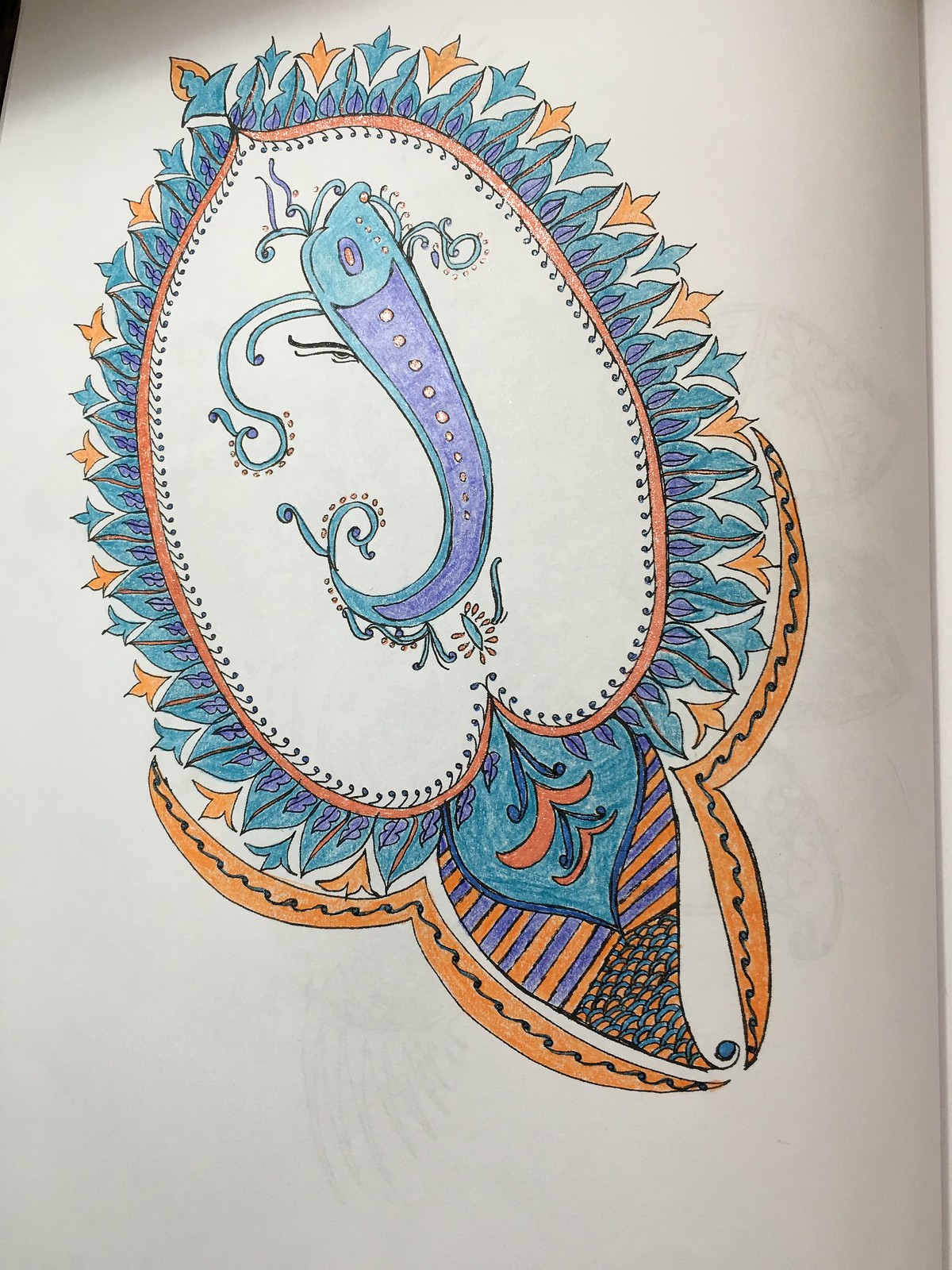The image captures a photo of an abstract, colorful pen and ink sketch drawn on what appears to be a sheet of slightly transparent, off-white or gray paper. The sketchbook page shows faint, overlapping lines from other drawings on the reverse side. The drawing features a central, enigmatic, organic shape that resembles an animal, potentially an axolotl, rendered in shades of purple and blue. Surrounding this central figure is a vibrant array of floral and leafy patterns, alternating in bright yellows, blues, oranges, and purples. The bottom section showcases striped designs in orange and blue, culminating in a border of orange with black squiggly patterns. The entire composition is set against a background that hints at a dark-colored surface peeking from the upper left-hand corner and a light-colored surface in contrast, emphasizing the sketch’s detailed and meticulous execution.